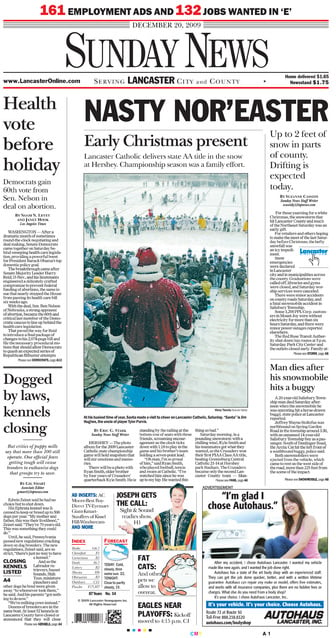**Sunday News - December 20th, 2009**

**Headline:** *Nasty Nor'easter Brings Early Christmas Present*

At the forefront of this edition is the image of a figure dressed in a Santa suit, viewed from behind, standing amidst a snow-covered stadium. The scene is set against a backdrop of heavy snowfall, with the entire stadium blanketed in snow, seats filled with spectators, and the field covered in white.

**Top Section:**
- **Employment Ads:** 161
- **Jobs Wanted:** 132 in E.
- **Domain:** LancasterOnline.com - Serving Lancaster City and County

**Above the Fold:**
- *Nasty Nor'easter:* The headline captures the severe weather event that has struck the region, leading to expectations of up to two feet of snow in parts of the county, with drifting anticipated throughout the day.
- *Early Christmas Present:* Accompanied by a photograph of a man in a Santa suit in the snowy stadium.

**Articles:**
- **Political Update:** Democrats secure their 60th vote from Senator Nelson regarding a deal on abortion, following a vote held before the holiday season.
- **Local Impact:** Due to stringent laws, several kennels are closing.
- **Tragic Incident:** A man loses his life after his snowmobile collides with a buggy.

**Additional Highlights:**
- **Weather Conditions:** Heavy snow and drifting predictions for the day ahead.
- **Human Interest:** A piece on "Joseph gets the call," featuring an image of a person, and another image of a woman in pink promoting, "I'm glad I chose Auto House," with the Auto House logo featured in the lower right corner.